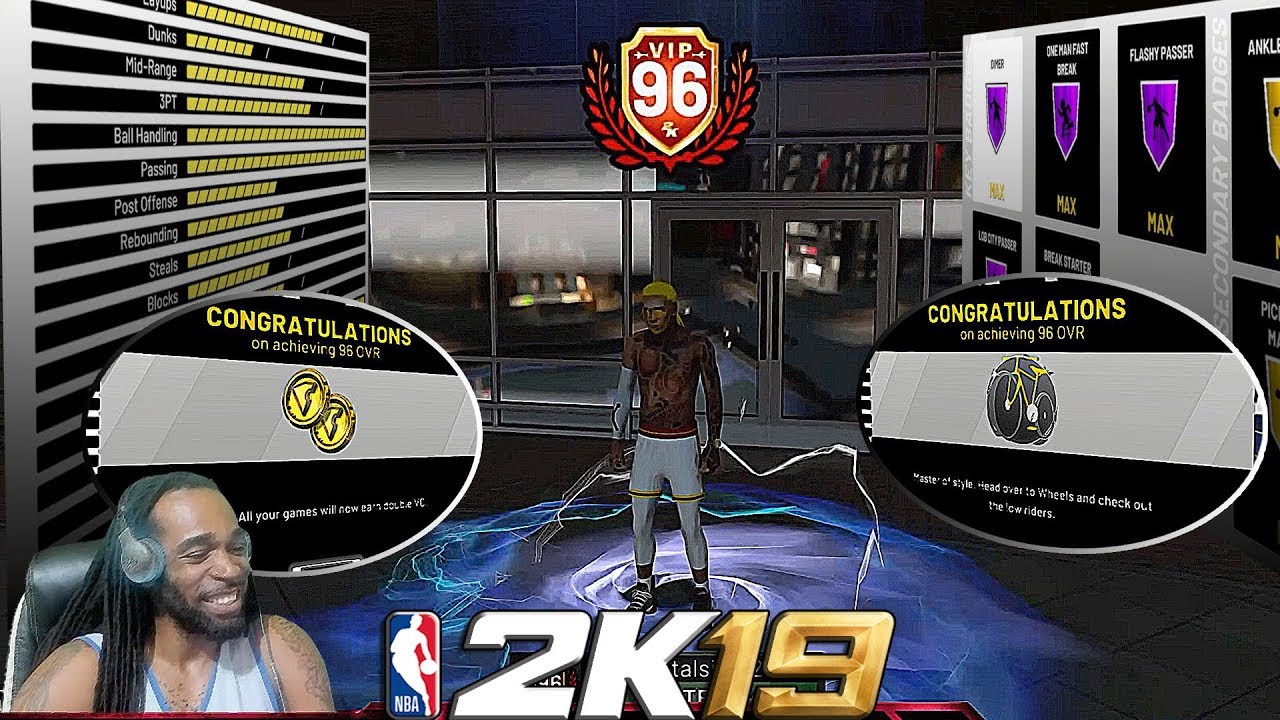Centered in the image is a detailed depiction of a video game character with a brown skin tone. The character appears shirtless, save for a garment or band wrapped around their left arm. They wear fitted jogger pants and tennis shoes, showcasing a modern, athletic look. Below the character, the text "2K19" is prominently displayed, with the NBA logo and the silhouette of a basketball player alongside the letters "NBA."

To the right of the character, a likely game vlogger is shown sitting in a tall, black gaming chair. He has black dreadlocks and is wearing a sleeveless shirt, smiling broadly with headphones on. Above his image is the phrase "Congratulations on achieving," accompanied by two gold coins beneath it.

On the left side of the image, a letter board is displayed, highlighting achievements of various players. The top center of the image features the title "VIP96," and to the right, the phrase "Congratulations on achieving 96QVR" is visible. Further right, additional player achievements are represented by purple diamond icons.

The background is animated, depicting a bustling cityscape from a video game. The scene includes a busy road flanked by tall, illuminated buildings, indicating a vibrant, nighttime urban environment.